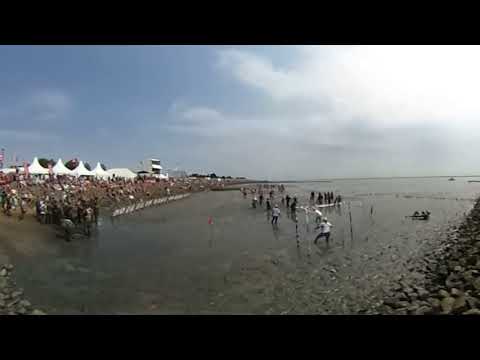This outdoor scene, possibly in a tropical setting and taken in the middle of the day, features several prominent elements framed by thick black borders at the top and bottom of the image. The foreground presents a murky brown body of water, extending from the center towards the right side of the image, where the shoreline and rocks are visible. Approximately 20 people, some wearing white shirts and most in black, are standing in the water, interacting with what appears to be a goalpost or obstacle. Directly above this, the sky transitions from blue in the upper right to grey clouds in the upper left. Off to the left of the water, further back, there are white-topped tents and clusters of people, suggesting a gathering or event. The overall setting gives the impression of an obstacle course or recreational activity near the water's edge, with the participants and onlookers contributing to the bustling scene.